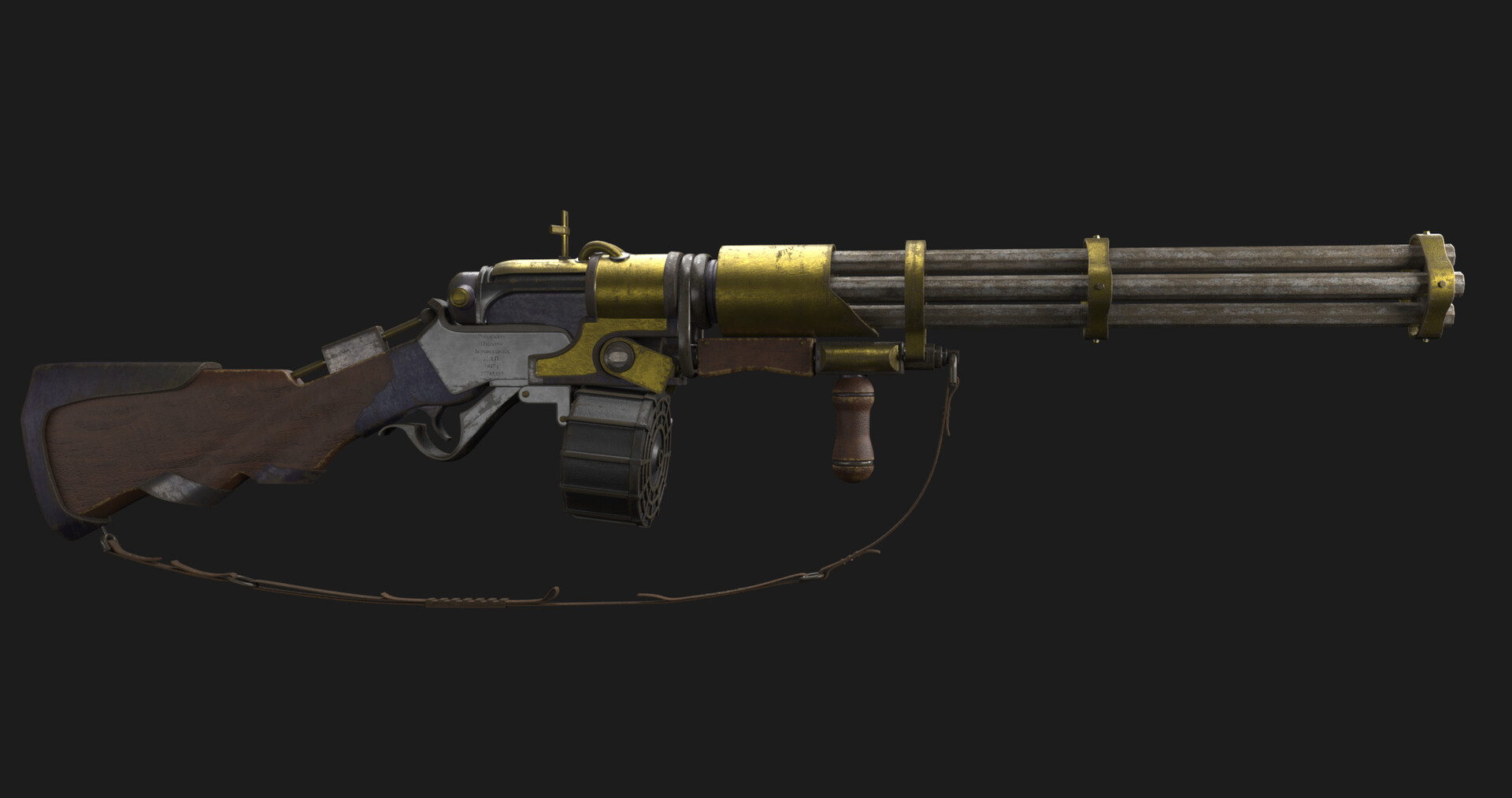The photograph showcases a meticulously detailed, old-fashioned steampunk gun set against a stark black background, making its features stand out vividly. The gun spans the width of the image, oriented horizontally from left to right. It possesses three to four long, silver barrels adorned with gold rings, giving it a weathered, yet ornate appearance. The gun's stock is made of wood and features a worn, brown leather padding designed to rest against the shoulder. A prominent, thin brown leather strap runs from the stock to the barrel's underpart. The trigger assembly is a striking silver, and some parts of the gun exhibit gold accents. Notably, the circular magazine or bullet carrier is positioned towards the front underside, suggesting an advanced yet anachronistic design, likely inspired by video game aesthetics. Overall, the gun exudes a futuristic steampunk vibe, blending elements of old craftsmanship with imaginative, game-like intricacies.